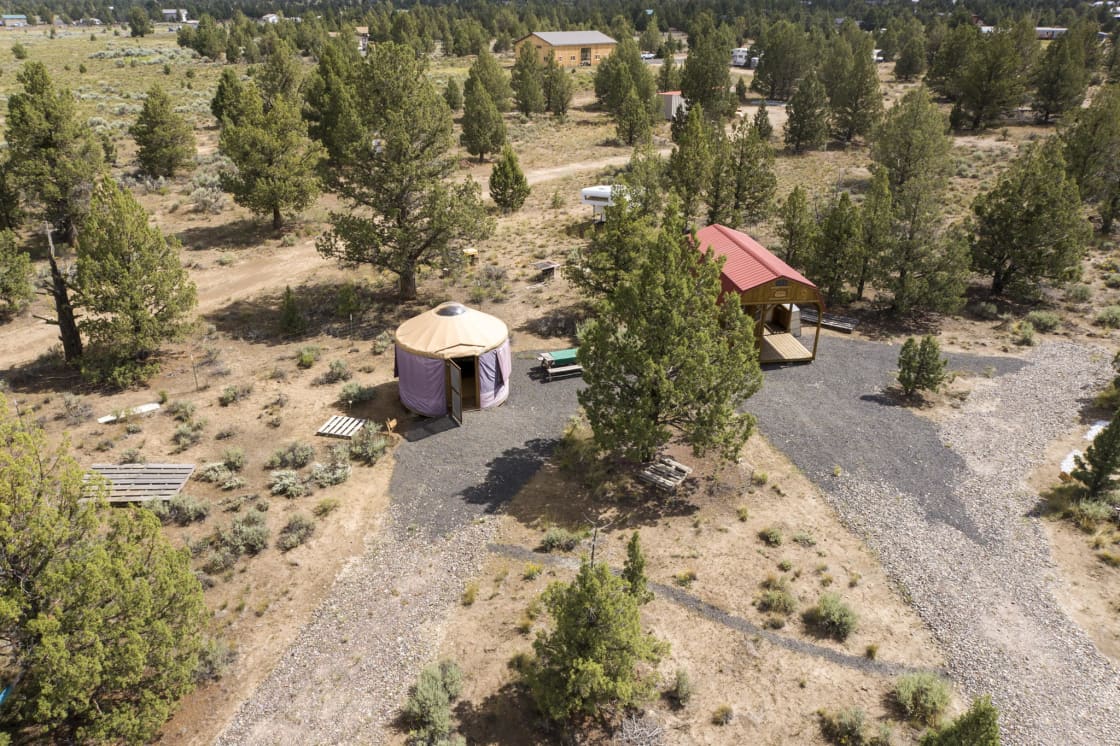An aerial view captures a serene woodland campsite, framed by dense trees with a sunlit ambiance. Central to the image is a U-shaped gravel road, with a large tree dominating the foreground and a smaller one in the backdrop. Adjacent to the road, a collection of structures suggest an active camping area. Foremost is a recently erected, grey domed tent-like structure, easily recognizable by its detachable design. Beside it stands a rustic wooden building with a wooden porch and a distinct reddish-pink roof. Further back, a small stable structure with a tan top and another yellowish house with a grey roof extend the campsite's layout. Scattered wooden planks lie on the ground, and in the distant background, cars and additional small houses, potentially farmland structures, are partially visible, indicating human activity and accessibility in the area. The setting exudes a lively yet tranquil atmosphere, perfect for an outdoor retreat.